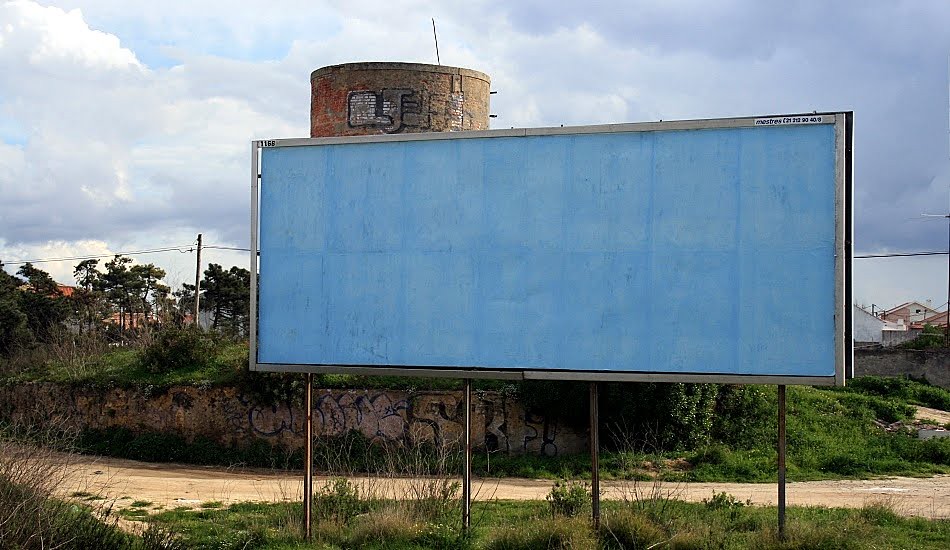This image depicts an outdoor scene during the daytime, characterized by a sky filled with clouds that dominate the upper and left portions of the photograph. Beneath the sky, the lower portion reveals a vibrant stretch of green grass interspersed with patches of beige dirt, hinting at a slightly uneven terrain that forms a small hill. On the right side, green plants and other vegetation are visible, adding to the lushness of the landscape. 

Centrally, there is a section of graffiti displaying a mix of yellow, white, and black hues. On closer inspection, some of the graffiti appears to include X-shaped marks, although these details remain somewhat indistinct. An unadorned billboard occupies a significant part of the middle ground; it features a light blue background devoid of any advertisements, suggesting that no commercial content has been placed on it as of yet.